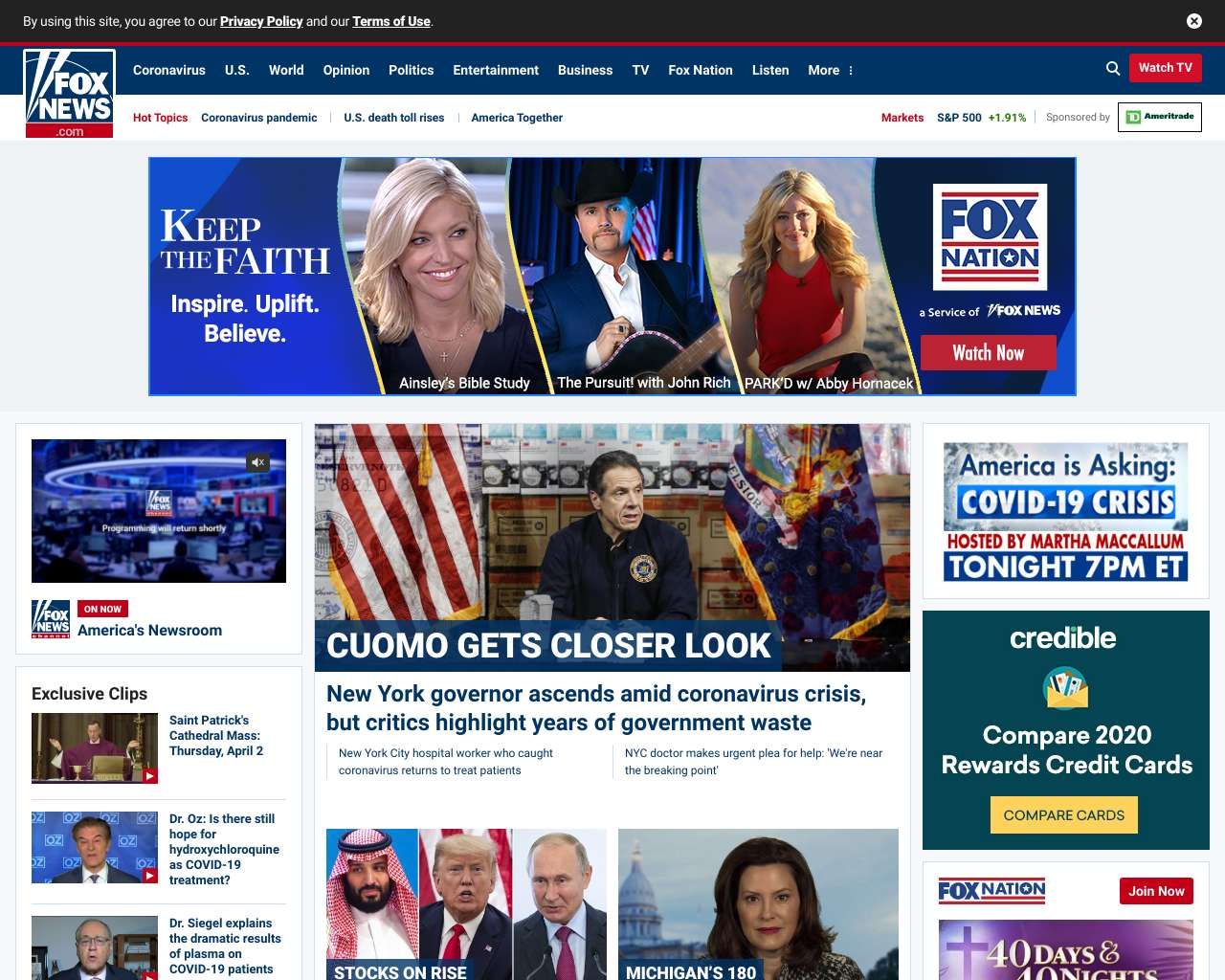This image captures the homepage of the Fox News website. On the left side, prominently displaying the iconic Fox News logo, which features two searchlights intersecting above a dome-like structure, with "FOXNEWS" emblazoned in bold white letters. Beneath the main logo text is a small rectangle that reads ".com" also in white.

At the very top of the page, there is a black bar with text that reads, "By using this site, you agree to our" followed by hyperlinked text for "privacy policy" and "terms of use" both in white.

Adjacent to the Fox News logo, a horizontal navigation menu features categories: Coronavirus, US, World, Opinion, Politics, Entertainment, Business, TV, Fox Nation, Listen, and a settings menu denoted by three dots. The 'Coronavirus' category is highlighted in red as a hot topic, followed by subcategories such as "Pandemic," "US Death Toll Rises," and "America Together."

On the right-hand side, there is a "Markets" section in red, showing the current status of the S&P 500 index with a green "+1.91" to indicate an increase, sponsored by Ameritrade.

A featured content segment includes a headline: "Keep the Faith, Inspire, Upload, Believe," with corresponding visuals of different anchors. One anchor, Ashley, is featured prominently, with her blonde hair and black dress or shirt, heading an event labeled "Ashley's Bible Study." Next to her, another image shows a cowboy figure in a white business shirt and dark blue tuxedo, holding an object. To the far right, there is a female reporter with long, shoulder-length hair in a strapless red dress, next to a bright red "Watch Now" button.

Below this segment, various news articles and updates are listed, focusing on COVID-related topics and other significant headlines, including a piece titled "Cuomo Gets a Closer Look."